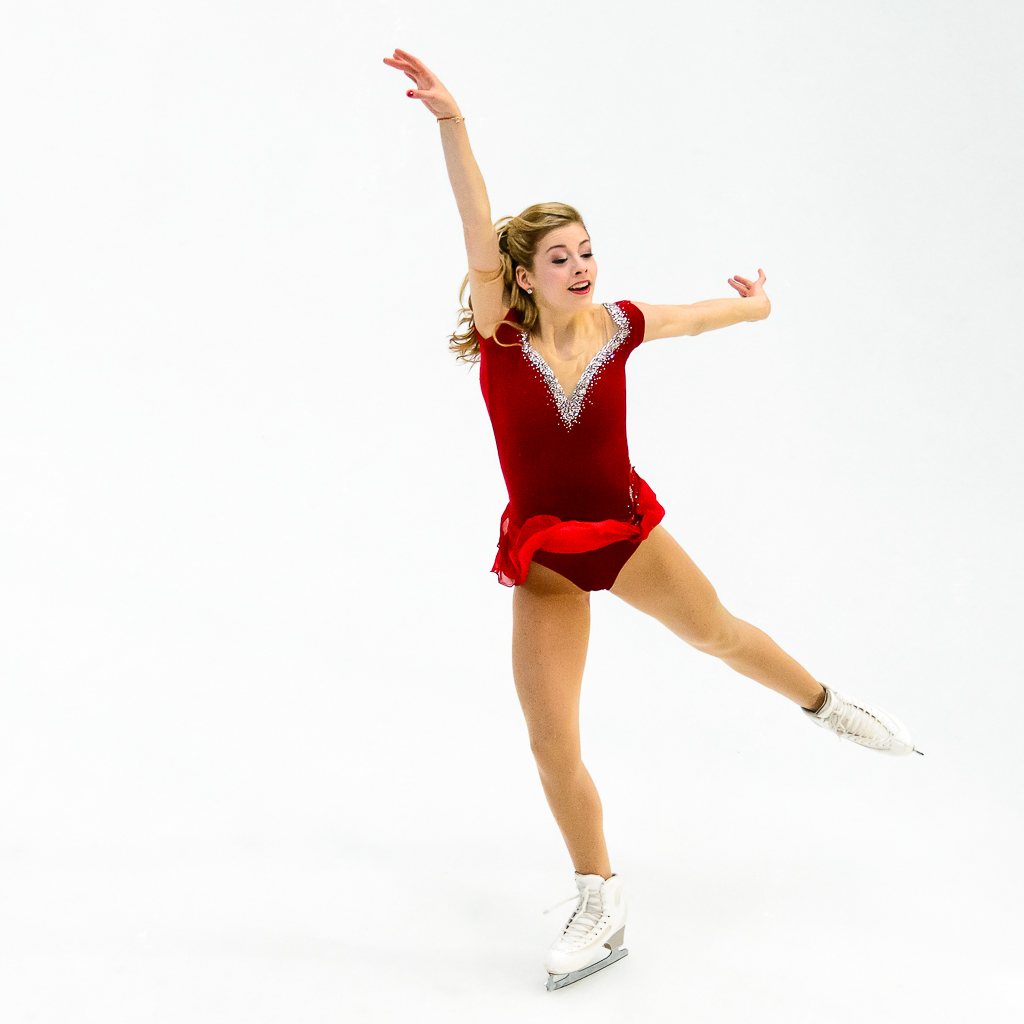In this photographic indoor image, a young white female ice skater is gracefully gliding across the ice. She sports white figure skates and is captured mid-performance, perhaps poised to take a jump. Her blonde hair is neatly tied back, and she wears red lipstick that complements her attire. The skater is dressed in a striking dark red velvet leotard with a flowing bright red accent skirt. The outfit is adorned with a sparkly silver collar. Her legs are stretched apart in an elegant pose; her left arm extends horizontally while her right arm reaches straight up. She accessorizes with red nail polish and a pair of earrings. The background is simple and grey, putting the full focus on her athletic beauty and poised grace.